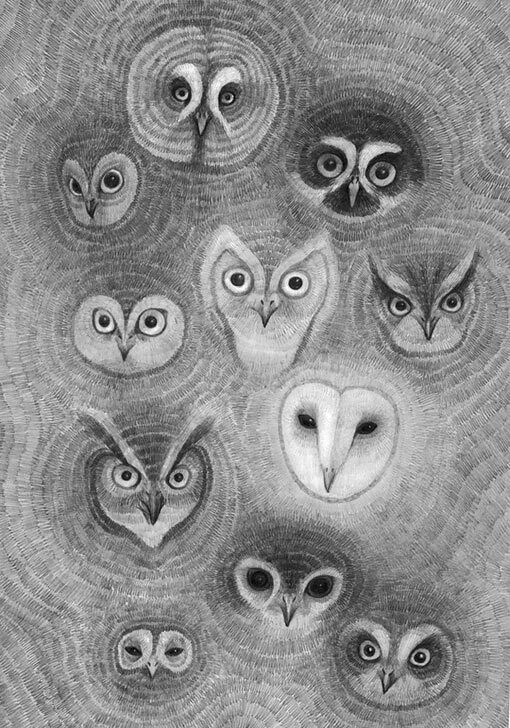This black and white pencil sketch illustration, reminiscent of a fabric print, features 11 distinct owl faces, each representing different species such as the iconic barn owl and the great horned owl with its prominent feather tufts. Arranged to cover the entire image, the owls’ faces are intricately detailed, focusing solely on their heads without depicting their bodies. Notably, the great horned owl near the bottom stands out with its distinctive feathered horns. The barn owl is also prominent, easily identifiable by its white heart-shaped face and black eyes. Other owls display unique characteristics, like the one in the top left with crescent moon patterns around its eyes and the ghostly white owl in the bottom right. Each owl features variations in eye shape, presence of eyebrows, and facial fur patterns, creating a mesmerizing array of avian visages all staring directly at the viewer.